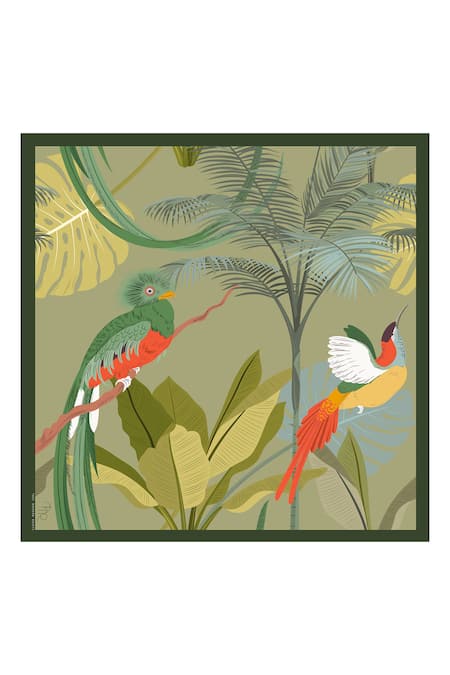This image showcases a detailed, Asian-influenced digital painting framed in a thin green border. The central background is a soft pea green, setting a tranquil tone. At the heart of the painting, lush tropical plants feature prominently, including long, teardrop-shaped leaves and palm-like branches extending from the bottom.

On the left side of the painting perches a striking bird with a vibrant green back and a red belly. Its head is adorned with green feathers resembling a small afro, and it has a yellow beak and bright white claws gripping a branch. The bird also displays a long, elegant green tail.

On the right, another bird with a slender, long beak appears mid-flight. This avian displays a varied palette with a gray neck, yellow breast, and a mix of white and green wings. Additional details include a black top of the head, red on the back of the neck, and a red tail, creating a striking visual contrast with the greenery around it.

The combination of intricate detailing in the birds and the lush plant life results in a rich, vibrant composition that feels both exotic and serene.